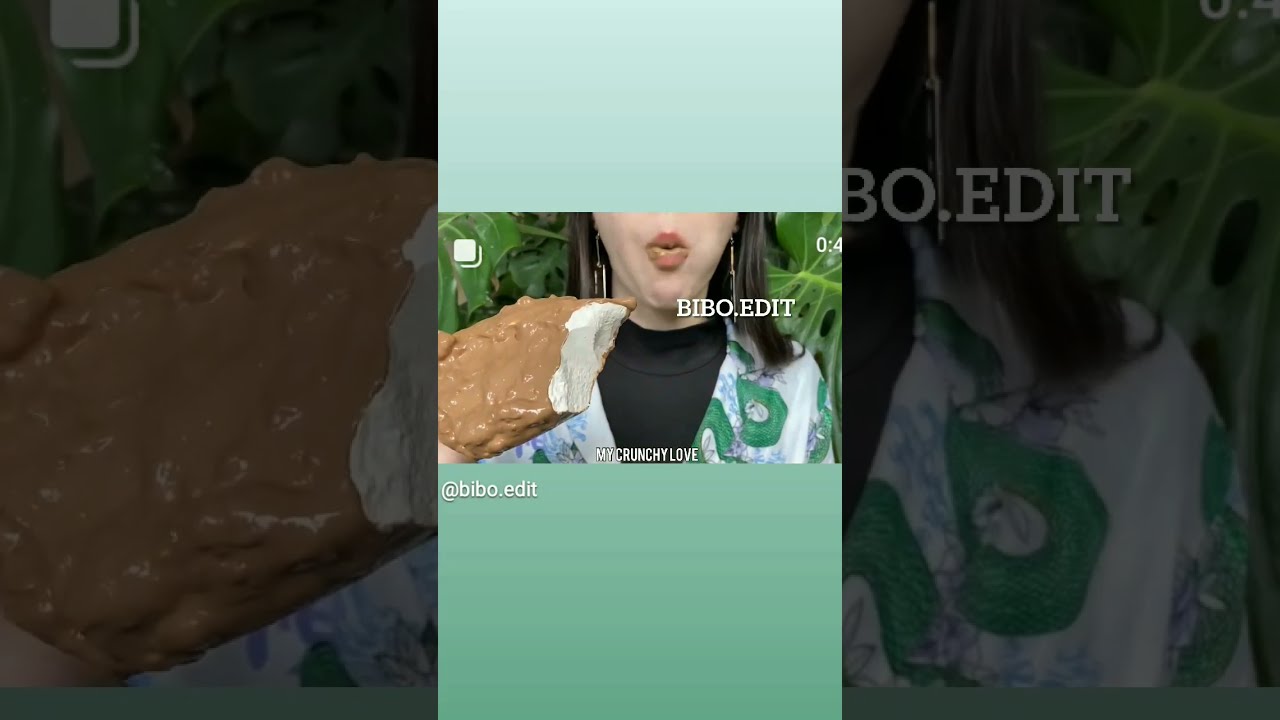In this photographic image, three panels present a detailed view of a woman and an ice cream bar. The central vertical rectangle, set against a light aqua background with darkened landscape borders, captures the woman from her nose to her chest. She is clad in a green and white floral jacket over a black mock-neck t-shirt, and she has long brown hair cascading over her shoulders. Her lips are puckered as she savors a chocolate-covered ice cream bar embedded with nuts. The background includes green leaves, enhancing the outdoor feel. The image text prominently displays "BIBO.EDIT" near her face and "My Crunchy Love" beneath the photo, with "@Bibo.edit" at the bottom. The image also features a time stamp "00:44". The left and right panels offer enlarged, grayscale close-ups: the left highlighting the crunchy ice cream bar, and the right focusing on her shoulder, hair, and part of her shirt with the text "Bibo.edit."